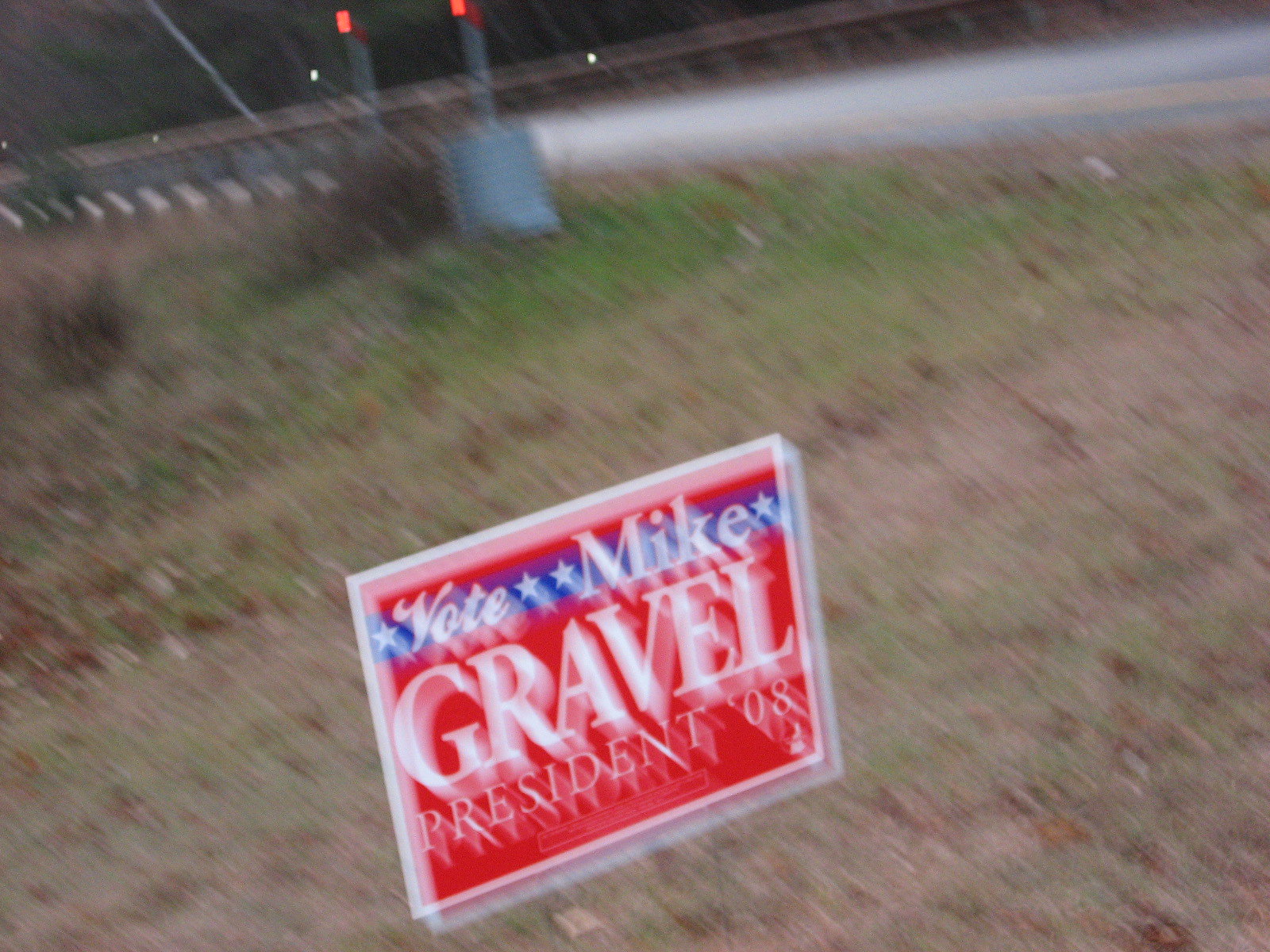In the foreground of this blurry outdoor image, patches of grass intermingle in hues of green and brown, indicative of both lively and dried segments. Scattered across the grass are numerous brown and tan leaves, giving the scene a sporadic, autumnal feel. Towards the front of the picture, a red and blue campaign sign is staked into the ground, emblazoned with "Vote Rebel President 08" in bold white letters. The background features a gray concrete asphalt road, along which a yellow or white line can faintly be discerned. Adjacent to the road, a series of metallic guardrails run parallel, contributing to the industrial ambiance. On the grassy roadside, a gray object lies partially visible amidst the blurriness, adding an element of mystery to the scene.